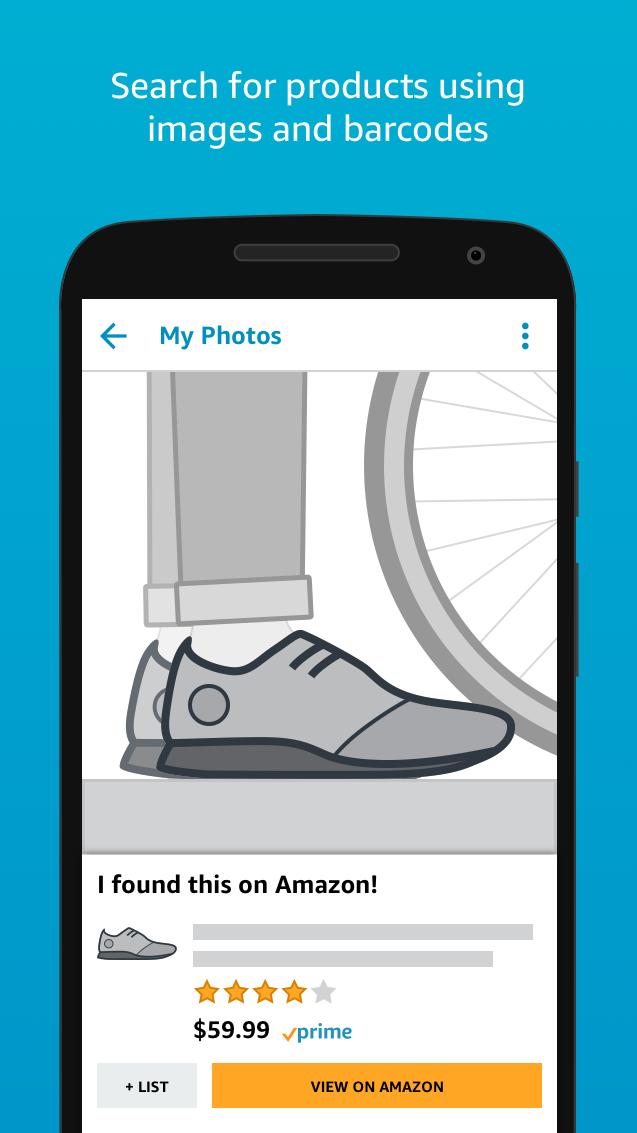In this detailed graphic artist's rendering or possible screenshot of a web page, the background color is a soothing baby blue. At the very top, a thin, water-colored font, which is prominently large but not overbearing, states: "Search for products using images and barcodes."

Below this text, there is an artistically-drawn close-up of a smartphone screen, simulating the Amazon app interface. At the top of the banner on the phone screen, there is a left-pointing blue arrow beside the phrase "This is my photos." 

In the main portion of the phone screen, the depiction showcases a side view of someone wearing gray pants and gray sneakers, with part of a gray bicycle tire visible in the background. This image represents the product being searched. The ground beneath is illustrated with a gray banner stretching from left to right. 

Beneath the product image and on the phone screen, black font text reads "I found this on Amazon." The text is accompanied by another smaller side view of the gray shoes, showing a rating of four out of five stars in yellow. Just below this, the price is displayed as "$59.99," and this is supplemented by an orange checkmark along with the word "Prime" in blue text.

Finally, an orange rectangular button at the bottom of the phone screen bears the text "View on Amazon" in black font, indicating a call to action for the viewer. This meticulous depiction vividly simulates a real-life Amazon browsing experience.